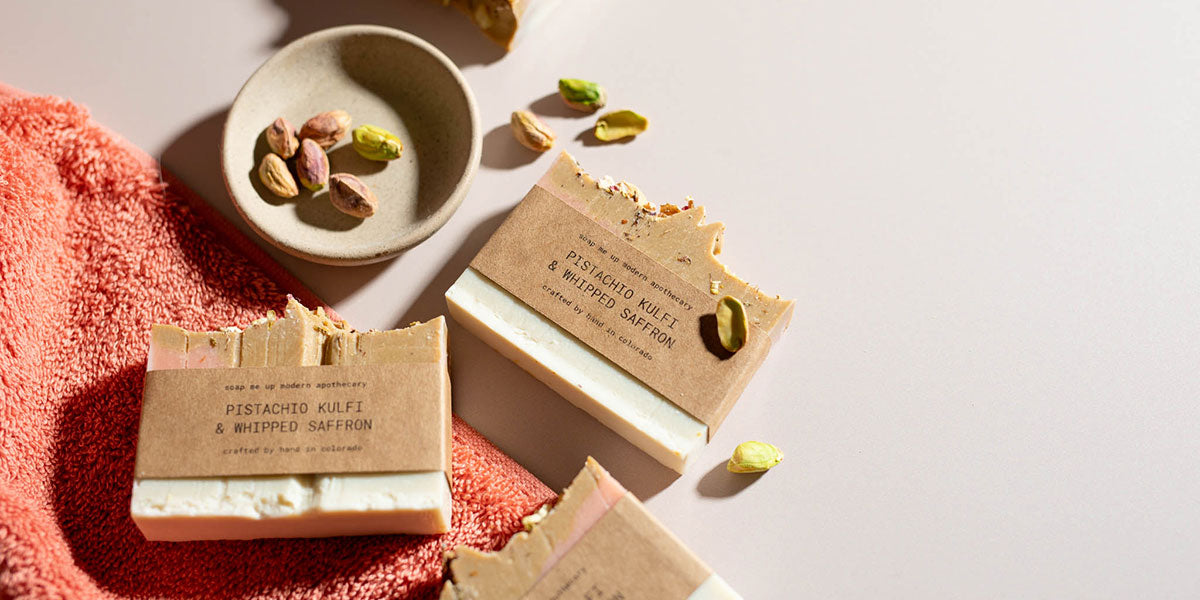The image features a detailed arrangement of candy and nuts set against a white background. In the lower-left corner, a melon-colored fuzzy towel serves as a base. Central to the image is a block of candy wrapped with a brown paper band labeled with "pistachio," "kulfi," and "whipped saffron," indicating these are the key flavors. The packaging suggests these come in bars, as the block shows signs of having pieces pulled off and partly eaten. There appear to be three bars included in a single package. Accompanying the candy is a small, cream-colored bowl situated in the upper left part of the frame, filled with shelled pistachio nuts, while a few loose shells—specifically three to five—are scattered around the base, enhancing the naturalistic presentation. The hand-crafted treats, made in Colorado, exhibit a rustic broken or bitten texture, emphasizing their artisanal quality.